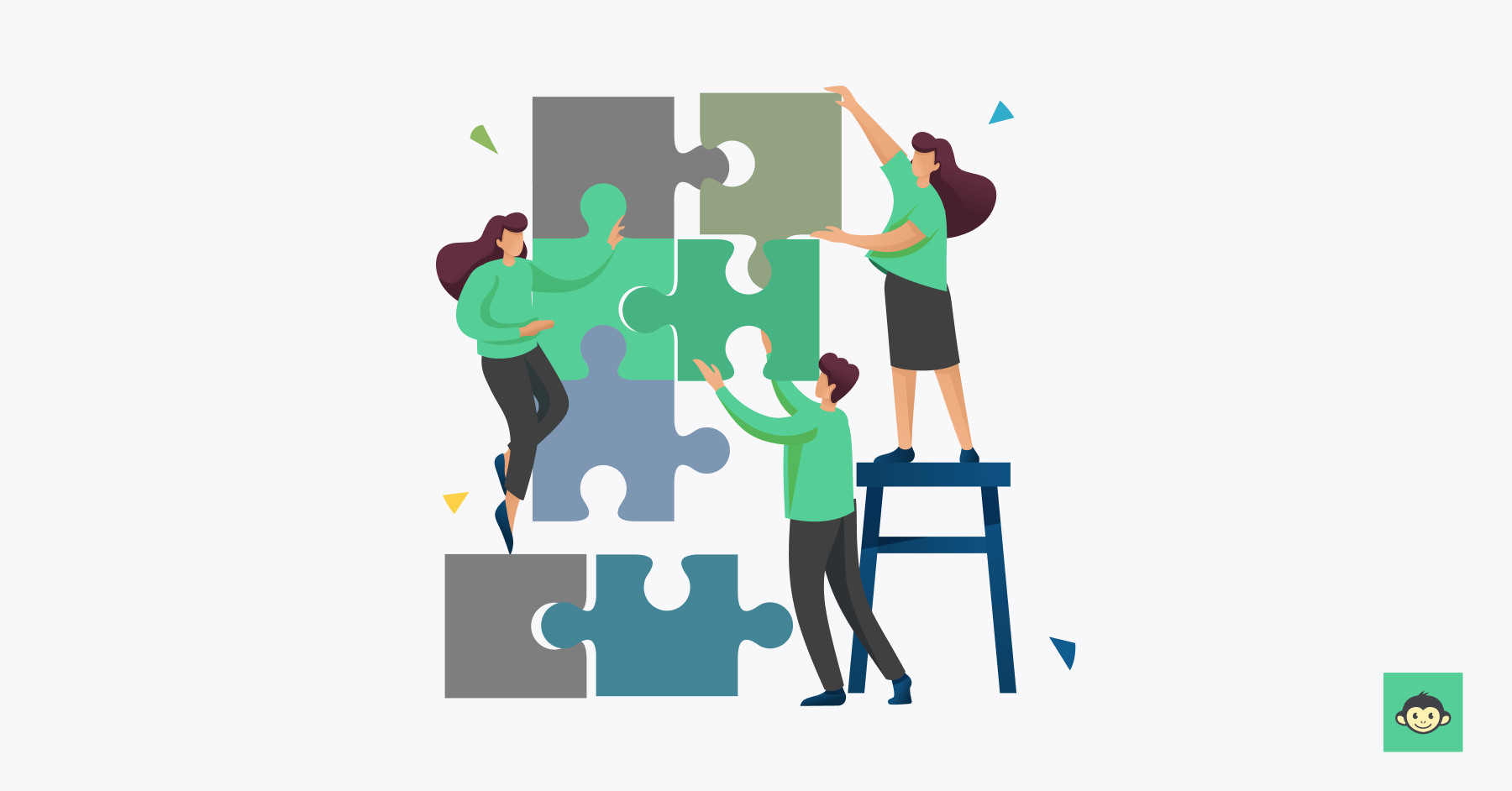The image is a vibrant, 2D illustration depicting three individuals, two women and one man, collaborating to assemble a large puzzle made up of various colored pieces, including sage green, light green, dark green, gray, purple, and teal. The woman on the right stands on a dark green stool, wearing a knee-length dark skirt and a Kelly green top, with brown, flowing hair. She reaches up to fit an olive-colored puzzle piece into place. Toward the bottom left, another woman with long dark hair, dressed in a green sweatshirt, leggings, and flats, is tiptoeing on a dark gray puzzle piece and directing her attention to another dark gray piece above, getting ready to connect it with the olive piece. The man, dressed in a green sweatshirt and black slacks, is positioned towards the bottom right, working to attach a dark green puzzle piece with a lighter green piece on the left. Below the assembled pieces, a teal puzzle piece and another bluish-gray puzzle piece are visible. In the lower right-hand corner, there is a small green square with a logo featuring a monkey's face. The illustration, characterized by its bright colors and simplistic graphic design without facial features, seemingly serves as a metaphor for collaboration and could be associated with themes like autism awareness.